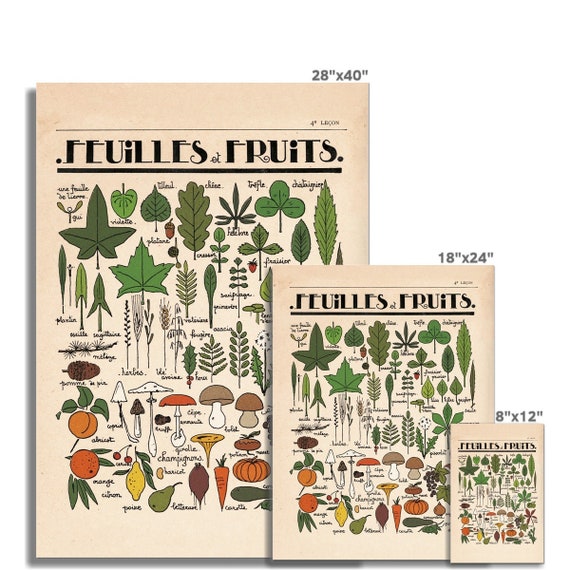The image showcases an educational poster available in three sizes: large (28 by 40 inches), medium (18 by 24 inches), and small (8 by 12 inches). The print features a detailed illustration of various fruits, vegetables, mushrooms, and leaves, each meticulously labeled with their names in a cursive, clipart-style. The upper section of the poster predominantly displays different types of leaves in vibrant green hues, progressing to a middle section illustrating various mushrooms, and concluding with a colorful array of fruits and vegetables at the bottom. This informative and visually appealing poster serves as both an educational tool and an attractive piece for décor, allowing you to learn and identify different plant species with ease. The dimensions of each available size are presented above the corresponding print, ensuring potential buyers understand the options.